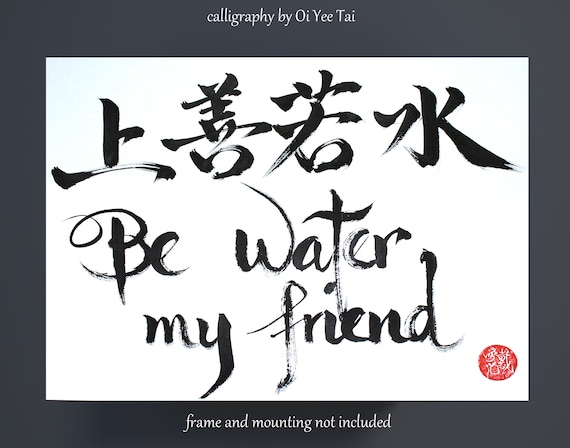The image features a white canvas bordered by a thick black mat. At the top of the mat, the text "Calligraphy by O-I-Y-E-E-T-A-I" is prominently displayed. Below this, in exquisite Japanese kanji calligraphy, there is a phrase rendered with visible brush strokes. This kanji is translated directly below into the English phrase "Be Water My Friend," written in an elegant, cursive style. In the bottom right corner of the canvas, a small red circle contains intricate white Asian characters. Along the bottom border of the mat, the note "Frame and mounting not included" is clearly printed. The overall composition is devoid of any human presence, allowing full focus on the text and calligraphy.